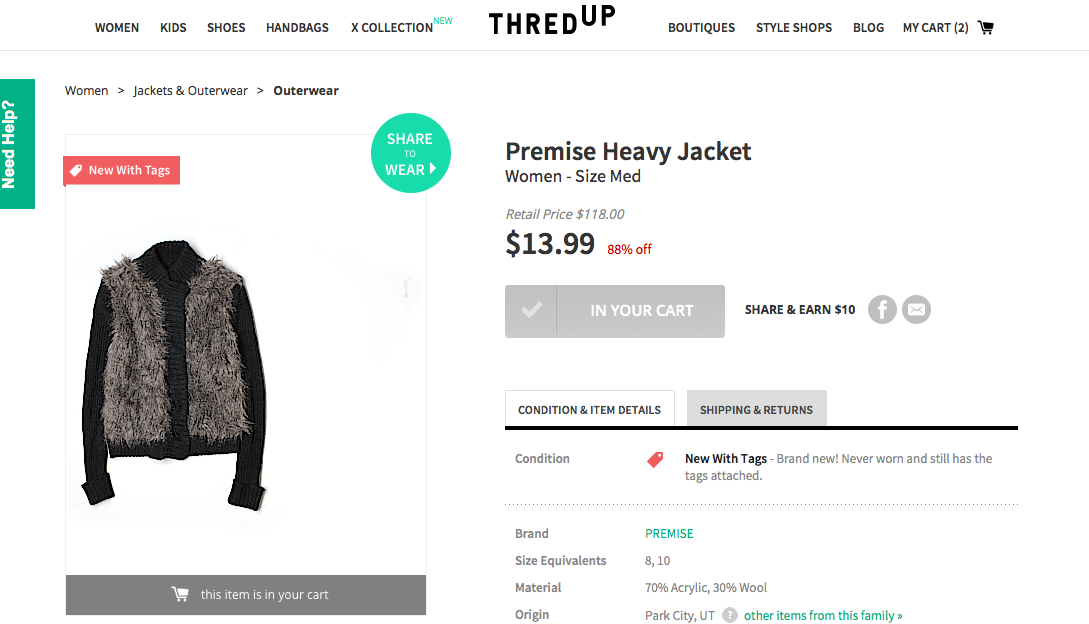Displayed on the ThreadUp website, this product page features a comprehensive view of a women's jacket prominently showcased. Across the top of the page, navigation tabs read: Women, Kids, Shoes, Handbags, and X Collection, with the larger ThreadUp logo followed by Boutiques, Style Shops, Blog, My Cart, and an image of a shopping cart.

The main product image presents a long-sleeved black jacket adorned with fluffy, fur-like portions on the front, embodying a blend of style and warmth. Above the image, the navigation path specifies: Women > Jackets > Outerwear.

Highlighted in red, the jacket is listed as "New with Tags." On the left, a green rectangle labeled "Need Help?" offers customer support.

The item description details the "Premise Heavy Jacket" in women's size medium. Retailing originally for $118.00, it is offered at a substantial discount of $13.99, which is 88% off. A check mark indicates the item is "In Your Cart," and prompts suggest "Share and Earn $10.00."

Further specifics state the condition as "New with Tags," meaning the item is brand new, never worn, with tags still attached. The brand is "Premise," with size equivalents of 8 and 10. The jacket is made of 70% acrylic and 30% wool, originating from Park City, Utah. A section below offers a link to "Other Items from this Family."